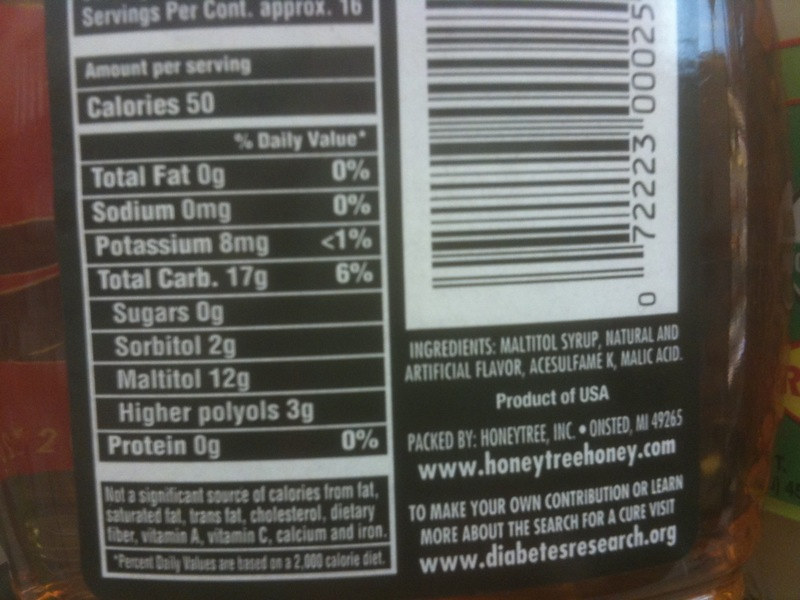This detailed color photograph captures a close-up view of part of a food label on a jar or carton. The label primarily appears in black and white, likely due to lighting or printing design. In the background, to the left, there are some red and black areas, hinting at other parts of the packaging or possibly another item. On the right side, the photo captures light reflecting off the container, revealing some colorful elements at the bottom, specifically green and red stripes.

The left side of the image features a blurred yet comprehensive nutritional facts table, listing various contents such as calorie content, fat content, sodium, potassium, carbohydrates, sugar, sorbitol, maltitol, and polyols including protein. The right side of the image shows a barcode set against a white background and some text outlining ingredients, including syrup, though not all of the text is legible. Additionally, it mentions the product is made in the USA and provides a website address: www.honeytreehoney.com.